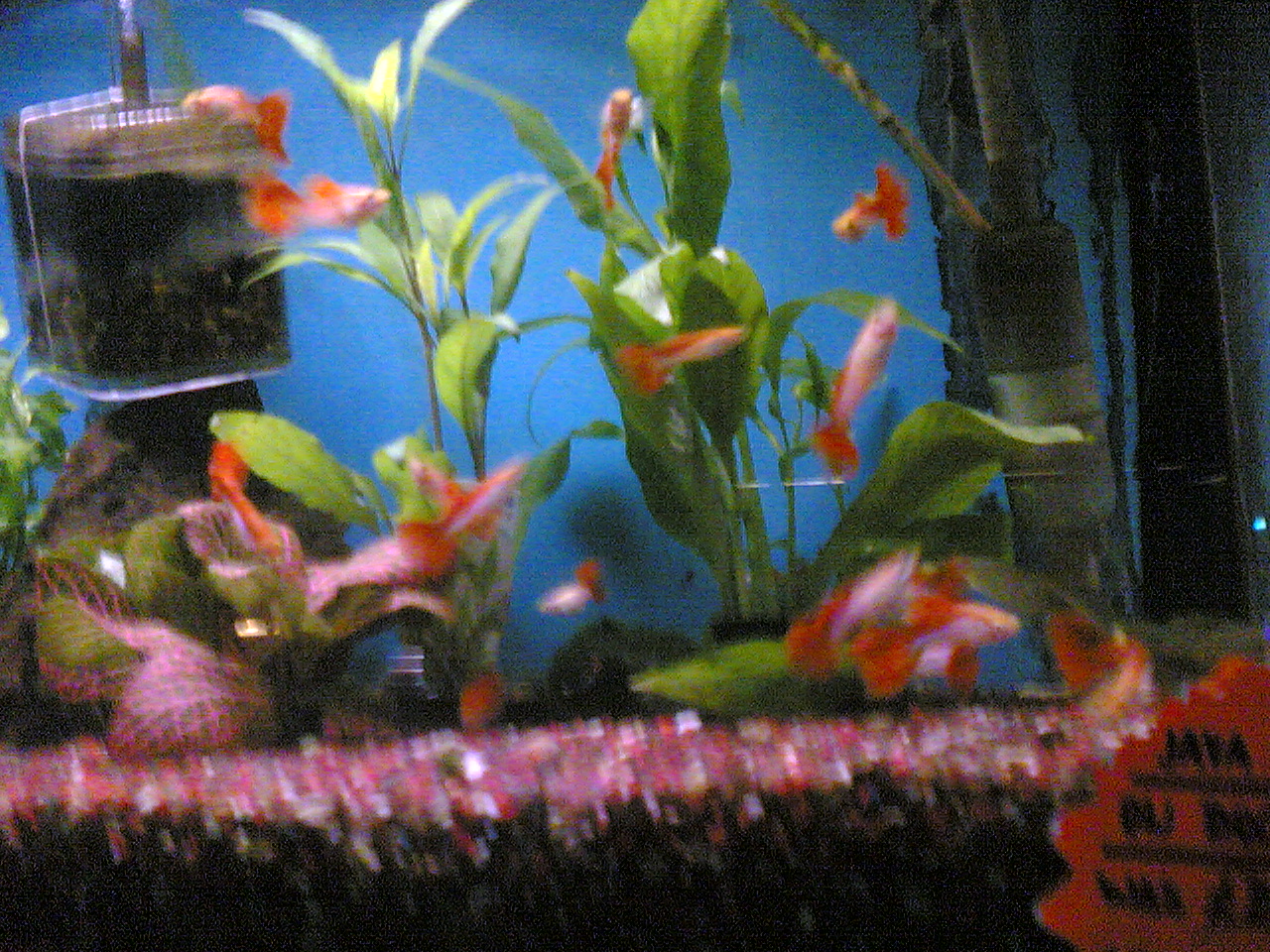The photograph is an out-of-focus image of a fish tank, likely taken in a pet store. The aquarium is populated with over a dozen small, orange and white fancy fantail goldfish. The tank's bottom is lined with gravel in shades of red, white, and brown, and features a mix of light green plants in the center and a green plant with pink vein lines on the left-hand side. Additionally, there is a black, glossy, round object on the left side of the aquarium floor. A filter is visible in the rear left-hand side of the tank. A small, orange starburst sign with barely legible black text is affixed to the front of the tank, further suggesting a pet store setting. Overall, the image is blurry and slightly tilted, obscuring finer details but clearly depicting the vibrant environment within the aquarium.